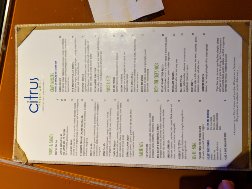A small, tilted image captures a menu from the restaurant "Citrus" laying sideways on a table. Although the text is unreadable due to the distance and size of the photo, the restaurant's name, "Citrus," is clearly visible in blue at what would be the top of the menu if oriented correctly. In the picture, this portion appears on the left side. The menu is densely packed with items, featuring two columns filled with a variety of offerings, all printed in small black type.